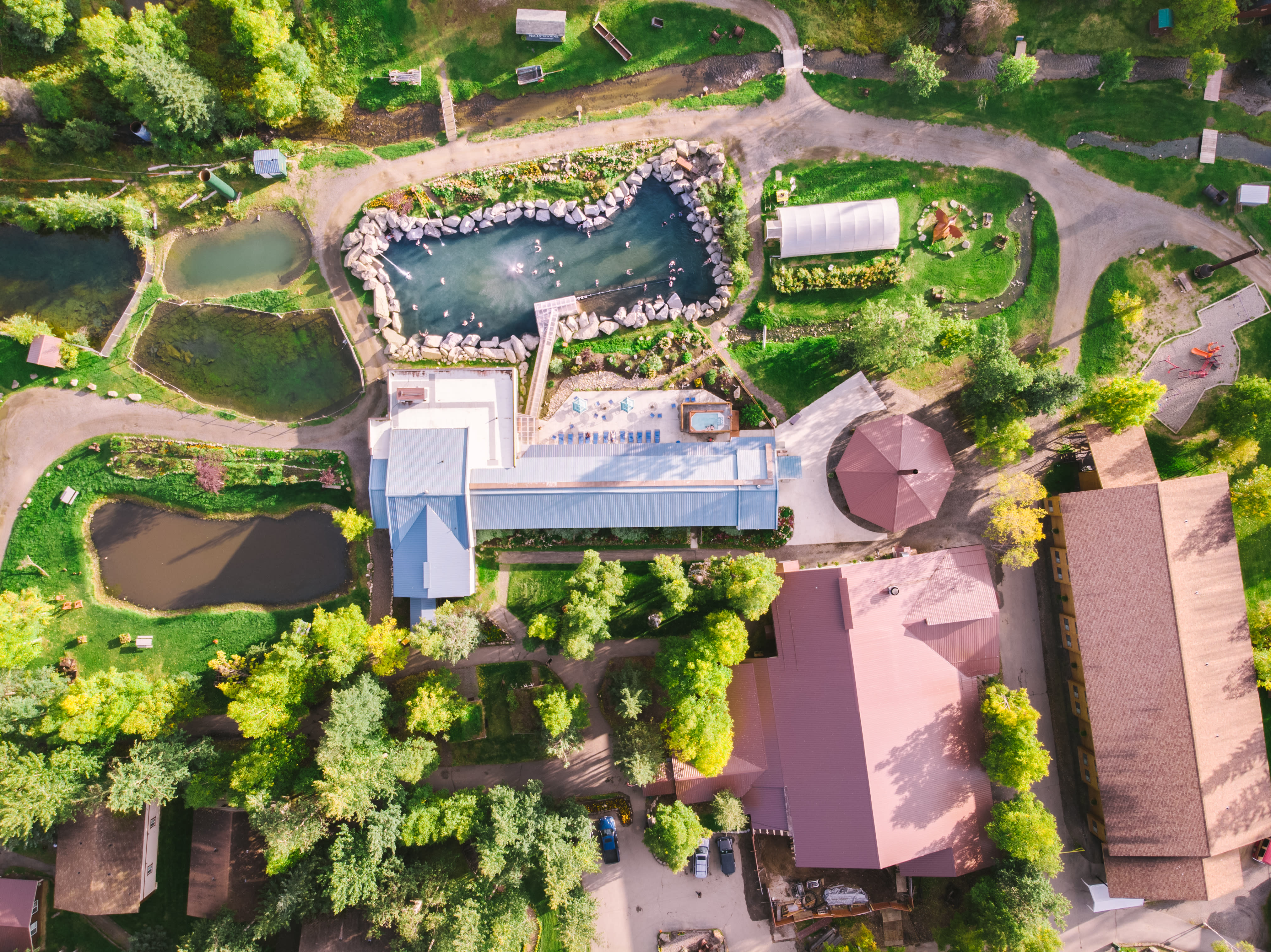This overhead aerial view depicts a diverse outdoor recreation area encircled by natural elements such as grass, brown dirt, and trees interspersed with beige sand or dirt pathways. Central to the interior is a large pond adorned with large gray boulders and characterized by its teal water, hinting at a possible fountain. Surrounding the pond are several white buildings, one notably featuring a reddish brick umbrella on its concrete patio. Scattered throughout are additional structures, some flaunting red roofs. To the front left of the image, smaller buildings are visible nearby the murky, brownish water body, suggesting another pool or pond. Further into the image, several cars are parked in front of one key building, enhancing the landscape with human activity. Trees and other areas with grassy plots or clearings contribute to the natural aesthetic of the space, completing this picturesque and multifaceted recreational ground.